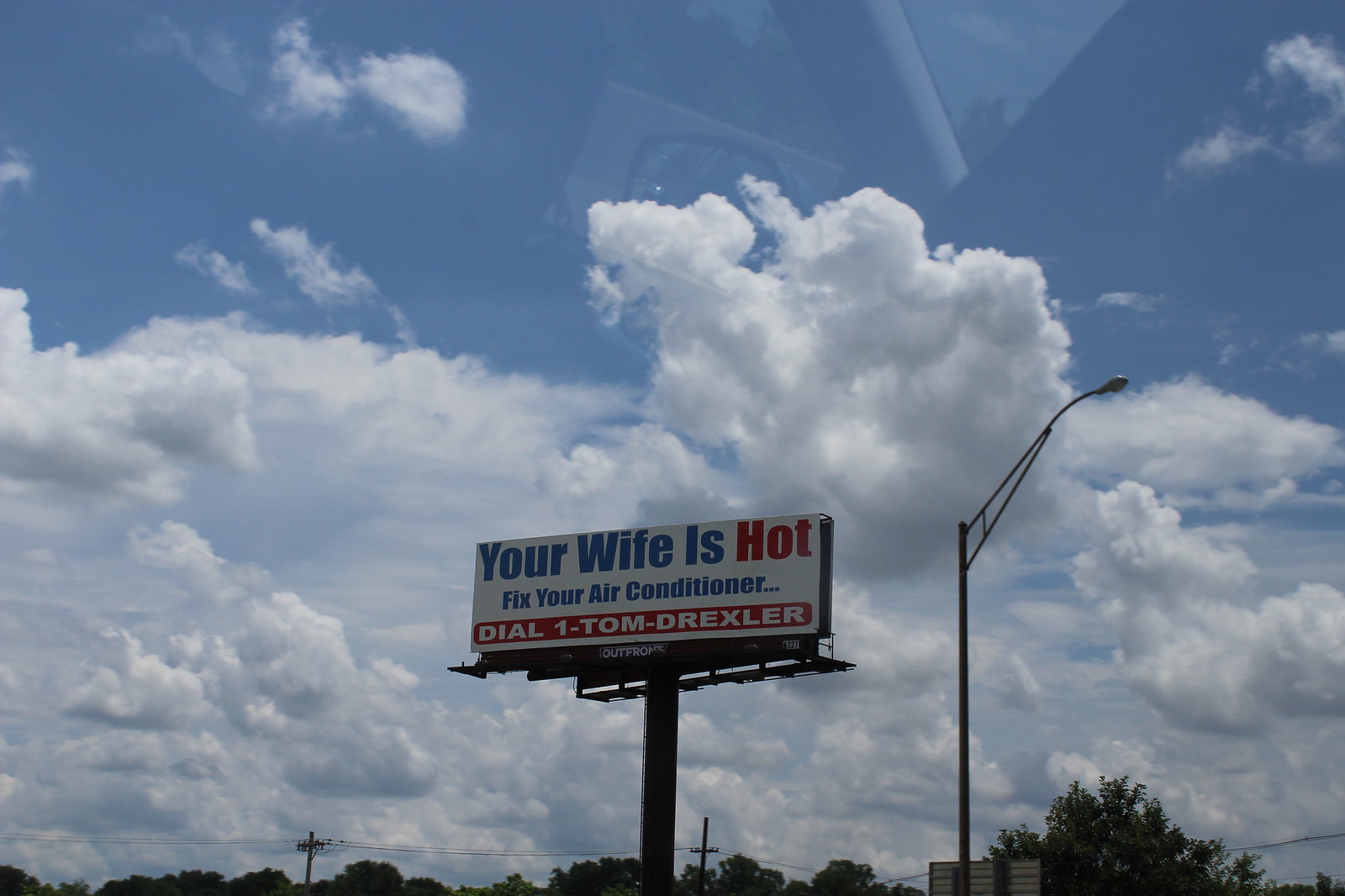The photograph depicts a tall billboard mounted on a large metal pole, positioned against a partly to mostly cloudy midday sky. At the top line of the billboard, bold blue and red text reads "Your wife is hot," followed by "Fix your air conditioner..." in smaller font. The call to action, "Dial 1-Tom-Drexler," appears at the bottom in red and white text. The billboard's background is white, contributing to its clarity and visibility. Surrounding the scene, power lines and green tree tops are visible at the bottom of the image. To the right of the billboard, an electric street light rises, possibly over a freeway. The sky features a mix of very fluffy, cotton-like white clouds and patches of bright blue, predominantly in the upper part of the photo. The image seems to have been captured from inside a car, indicated by the faint reflection of the car’s interior on the window.